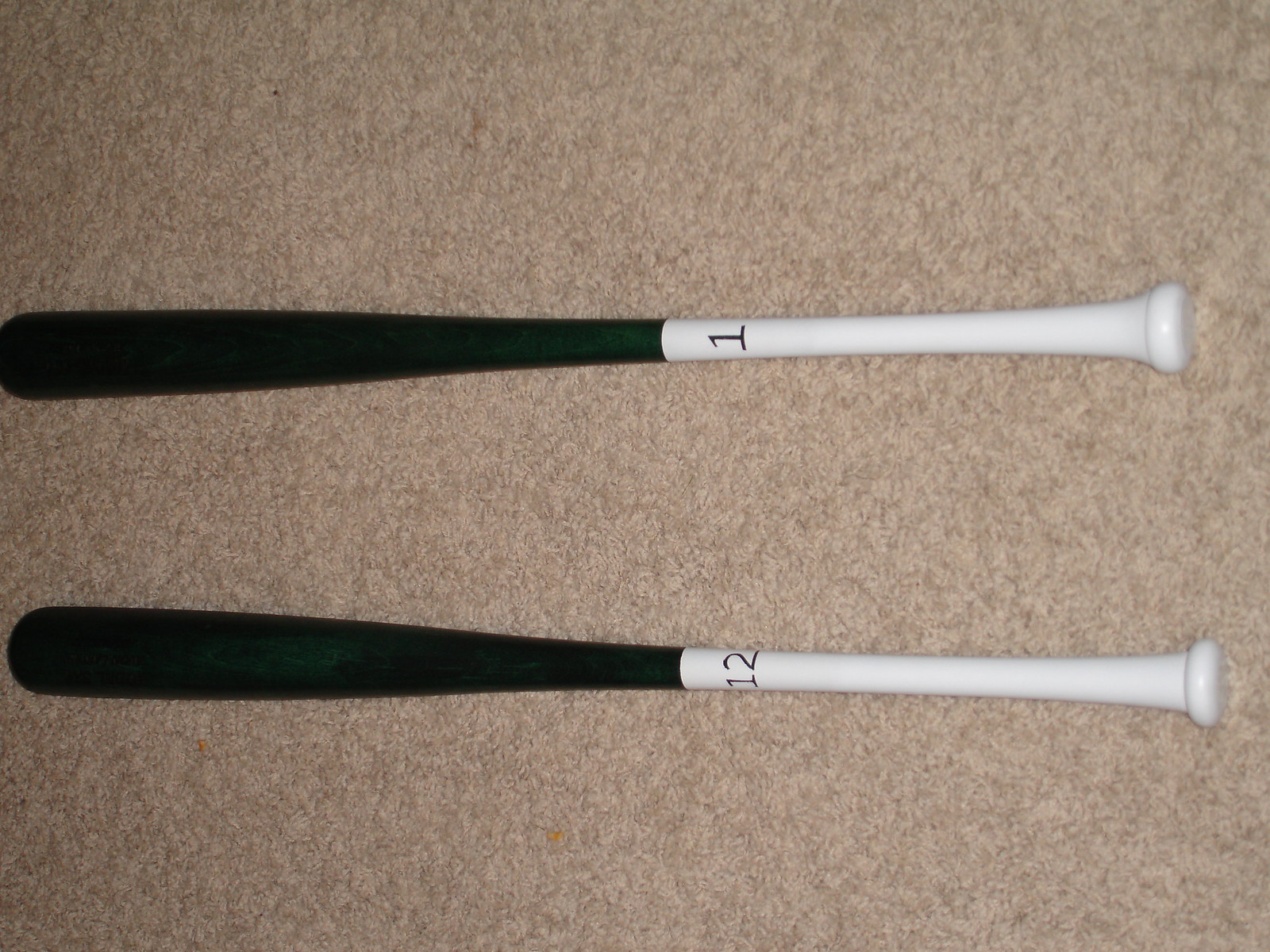This is a high-quality color photograph taken from above, showcasing two baseball bats placed horizontally on a beige, mottled carpet. The bats, positioned one on top of the other with about a foot and a half between them, feature matte black tops and pure white handles where they are gripped. The bat on top is marked with the number 1 in black, while the bat on the bottom is labeled with the number 12, also in black. The overall image captures the sleek, minimalist design of the bats against the textured carpet background, suggesting a deliberate and well-composed scene, possibly for a sale or personal collection display.